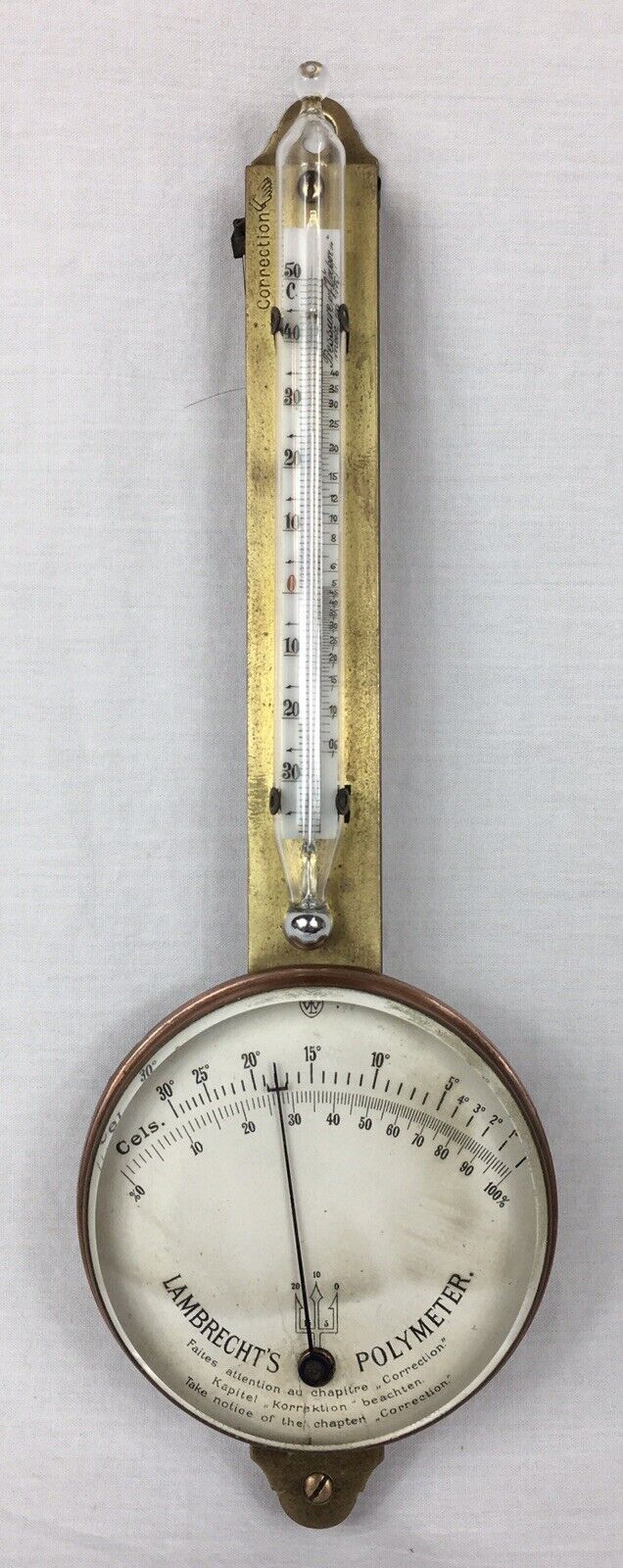This image features a vintage brass and brown Lambrichts Polymeter, mounted vertically against an ivory-colored background. The device is a multipurpose barometer with a round face displaying various readings. A long, narrow arm with a pointed tip extends from the center of the circle, used for measuring temperature in both Fahrenheit and Celsius. The thermometer tube is secured with brackets and appears to be mounted with screws on the wall. The dial is bordered with additional non-English text in black, contributing to its intricate and aged appearance. At the base of the circle, "Lambrichts Polymeter" is clearly inscribed, giving the instrument an air of historical significance. This piece closely resembles a combination of a temperature gauge and a clock, providing a detailed, multifaceted reading of environmental conditions.